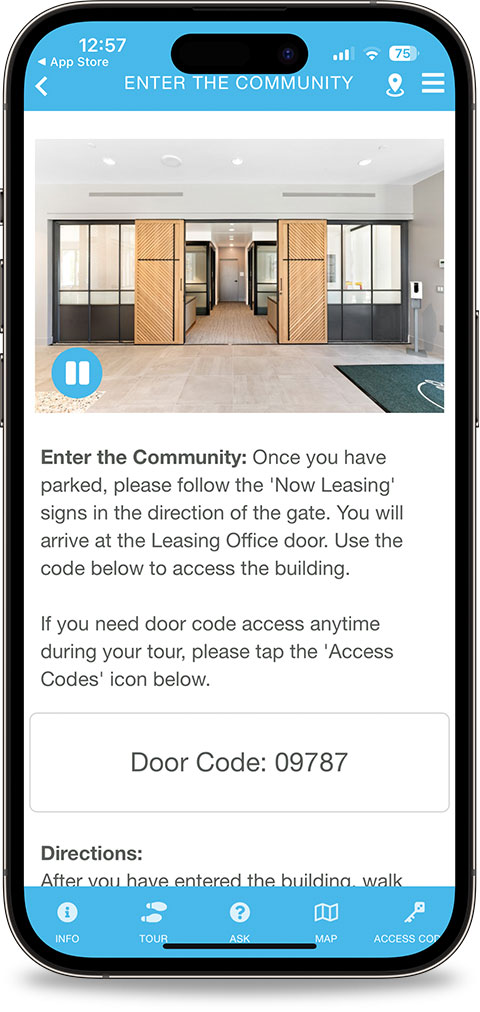The image is a screenshot of a smartphone displaying an app. At the very top, there are standard indicators such as the time, Wi-Fi signal strength, and battery percentage. Beneath this, a navigation bar features a white back arrow, labeled "App Store," alongside a location button on a blue background. 

The main content starts with a header image depicting a lobby area with wooden doors, wooden flooring, and a green carpet. Below the image, text reads, "Enter the community. Once you have parked, please follow the now leasing signs in the direction of the gate. You will arrive at the leasing office door and use the code below to access the building. If you need door code access anytime during your tour, please tap the Access Codes icon below, and the door code is 09787."

Underneath, there is a section titled "Directions," with the instruction starting, "After you have entered the building, walk..." but the text is abruptly cut off.

At the bottom of the screen, icons on a blue background provide additional options: "info" with an 'i' icon, "tour" with two hands icon, "ask" with a question mark icon, "map" with a map icon, and "Access Code" with a key icon. The screen primarily features a white background with black text and blue borders.